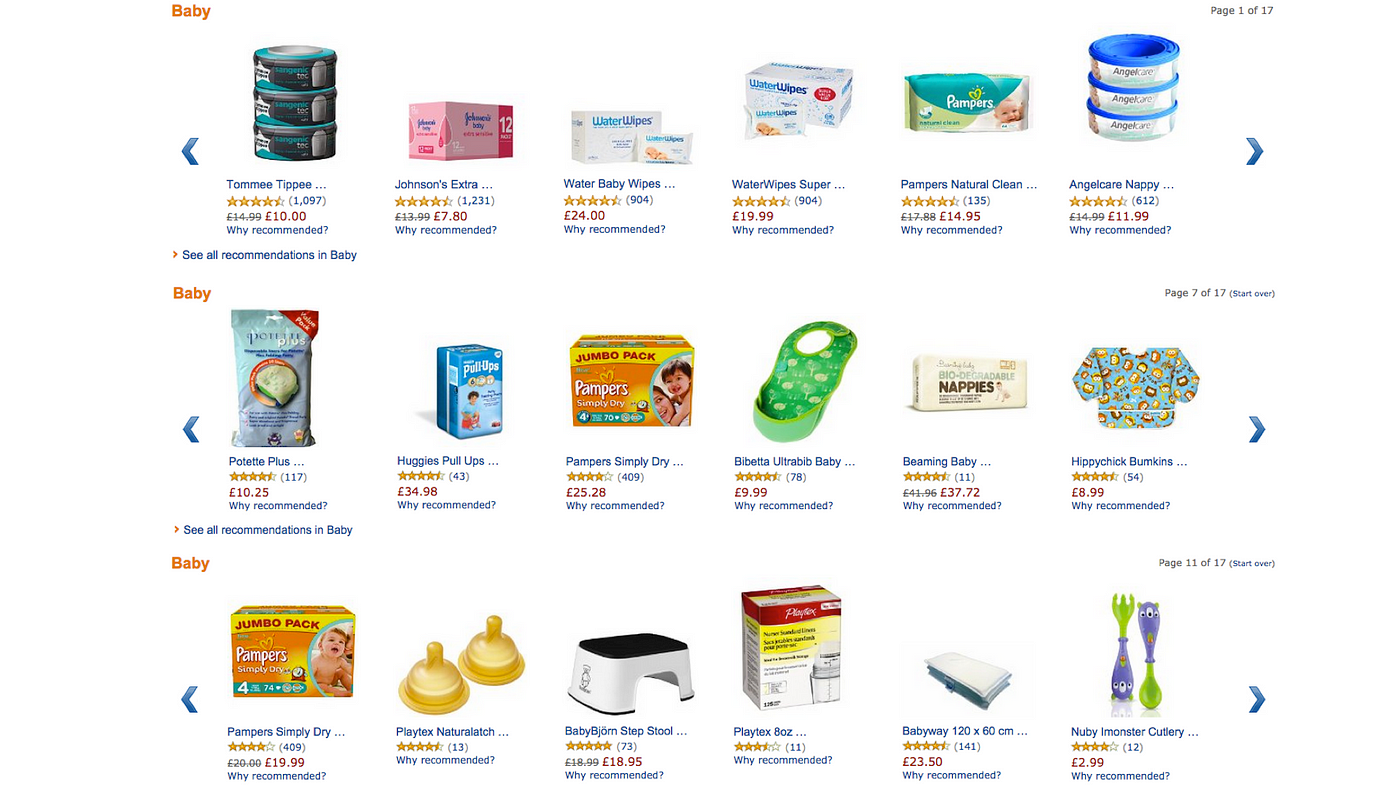The image depicts a web page designed for purchasing various baby products. The layout is organized into three distinct rows, each featuring six different items accompanied by their respective prices and reviews, including star ratings and the number of reviews.

In the first row:
1. The first item is labeled "baby" and appears to be a stack of three cans.
2. The second item is Johnson's Extra Baby Powder, presented in a pink box.
3. The third item is Water Baby Wipes.
4. The fourth item is a larger container of Water Wipes Super.
5. The fifth item is Pampers Diapers.
6. The sixth item is Angel Care Nappy disposal system.

In the second row:
1. The first item is a packaged baby food product.
2. The second item is Huggies Pull-Ups training pants.
3. The third item is a Pampers Jumbo Pack of diapers.
4. The fourth item is an Ultra Bib for Babies, colored green.
5. The fifth item is a pack of Biodegradable Nappies.
6. The sixth item is another Jumbo Pack of Pampers.

In the third row:
1. The first item is a Jumbo Pack of Pampers diapers.
2. The second and third items are different types of nipples for baby bottles.
3. The fourth item is a step stool.
4. The fifth item, labeled Playtex, is an 8-ounce container for baby bottles.
5. The sixth item is a set of what appears to be sheets or a crib mattress, branded as Baby Way.
6. The last item is Nubby Eye Monster Cutlery, designed for kids.